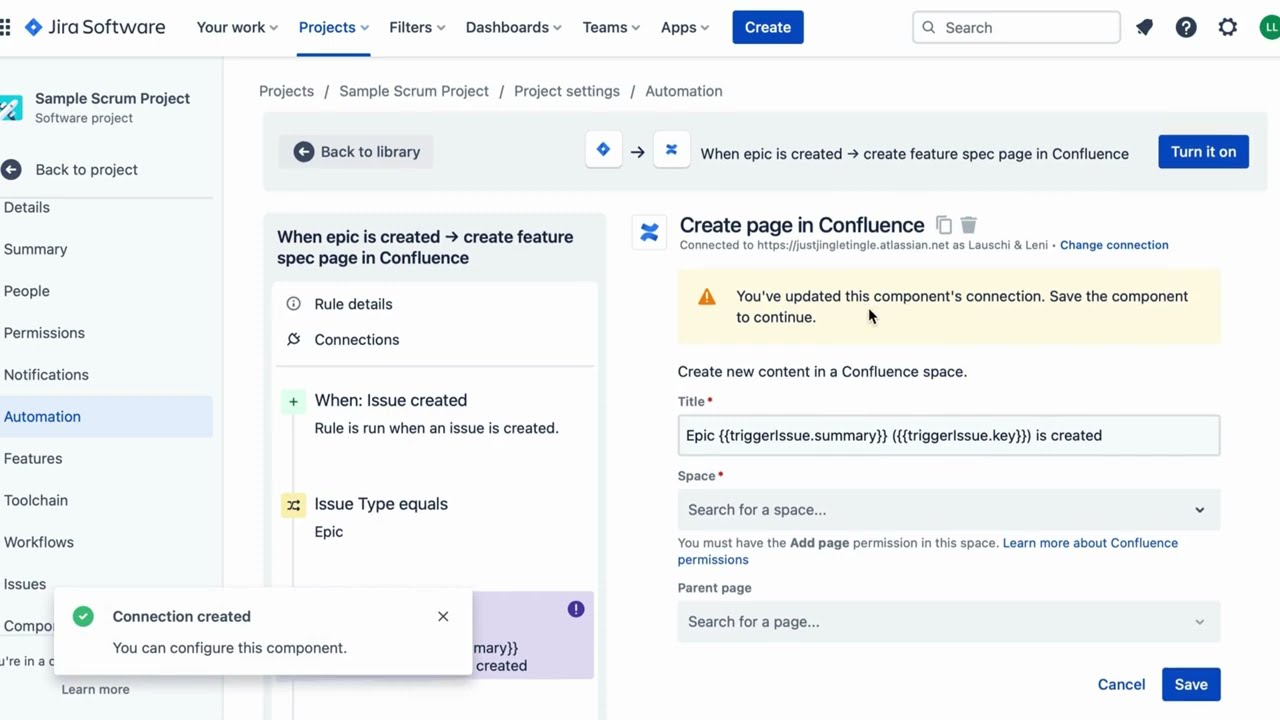The image shows a detailed dashboard for JIRA software. On the upper left corner, the JIRA logo, a blue diamond shape, is prominently displayed alongside the text "JIRA software". To its right, a horizontal menu bar includes options such as "Your work", "Projects", "Filters", "Dashboards", "Teams", "Apps", and a blue "Create" button. This menu also features a search bar with a magnifying glass icon, and several notification icons including a bell, a question mark in a circle, a cog wheel, and a green circle with the user's initials "LL".

Below this menu, the screen is divided into sections. The left-hand column, shaded in light gray, lists options vertically: "Sample scrum project", "Software project", "Details", "Summary", "People", "Permissions", "Notifications", "Automation", "Features", "Toolchain", "Workflows", and "Issues". At the bottom, a message with a green checkmark reads "Connection created. You can configure this component".

To the right, another column displays a header "When Epic is created, create feature spec page in Confluence". Underneath, there's some additional text and warnings, such as "You've updated this component's connection. Save the component to continue". The background is predominantly white, with text in shades of gray and black, while various buttons such as "Cancel" and "Save" are also present. The overall layout indicates this is a screenshot from a computer, used to manage projects and workflows within JIRA software.